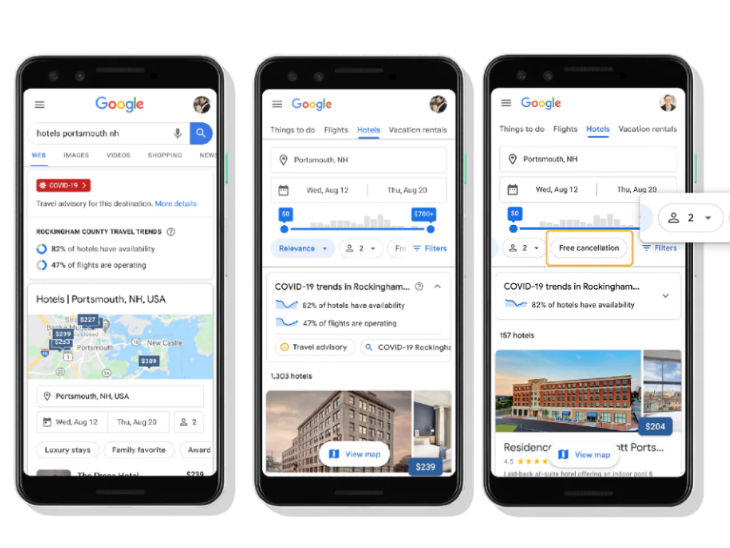The image showcases three distinct smartphone screens, each displaying Google search results. The screens have black edges at the top and bottom, framing a predominantly white background with various search information. 

On the leftmost screen, the search query "Hotels Portsmouth NH" is entered. Below the search bar, there are results featuring COVID-19 updates for Rockingham County, a map of Portsmouth, NH, and visual price markers represented as blue squares. Further down, the screen displays another link titled "Portsmouth NH COVID-19 trends" accompanied by an image of a building.

The middle and rightmost screens differ slightly, with both searches refined to focus on "Hotels." Each screen has a date range indicated as "Wednesday, August 12th to Thursday, August 29th," followed by a price range bar. Both screens under the 'Hotels' section display another image of a building within Portsmouth, NH. The middle and right screens are specifically highlighted under the 'Hotels' tab, as indicated by the section being blue, while the leftmost screen is highlighted under the 'Web' tab.